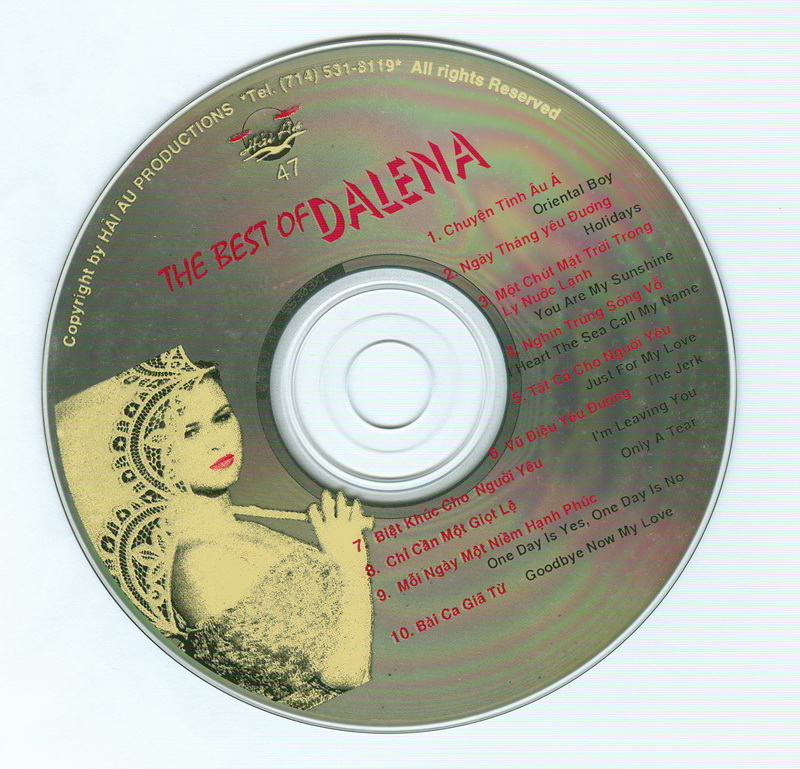This is the front of a compact disc titled "The Best of Delina." The disc has a metallic gold color accented with red, black, and white elements. Prominently featured on the left side is a striking image of a woman wearing a low-cut blouse that exposes her shoulders, along with bright red lipstick and black eyeliner. She holds a lacy umbrella, adding a touch of elegance and vintage charm to her appearance.

At the top of the disc, in small yellow lettering, is the text: "Copyright by Hey Al Productions, telephone number 714-531-8119, all rights reserved." Above this, there is a tiny logo featuring the number 47 and the name Hi Ah, which includes a circular design with red wings and intricate details involving a bird and some text.

The title "The Best of Delina" is written in red on a slant at the top left of the disc. The tracklist, presented in both English and another language, runs from the upper right down to the center of the disc, listing ten songs: 1. Oriental Boy, 2. Holidays, 3. You Are My Sunshine, 4. I Heart The Sea, 5. Call My Name, 5. Just For My Love, 6. The Jerk, 7. I'm Leaving You, 8. Only A Tear, 9. One Day Is Yes, One Day Is No, 10. Goodbye Now, My Love.